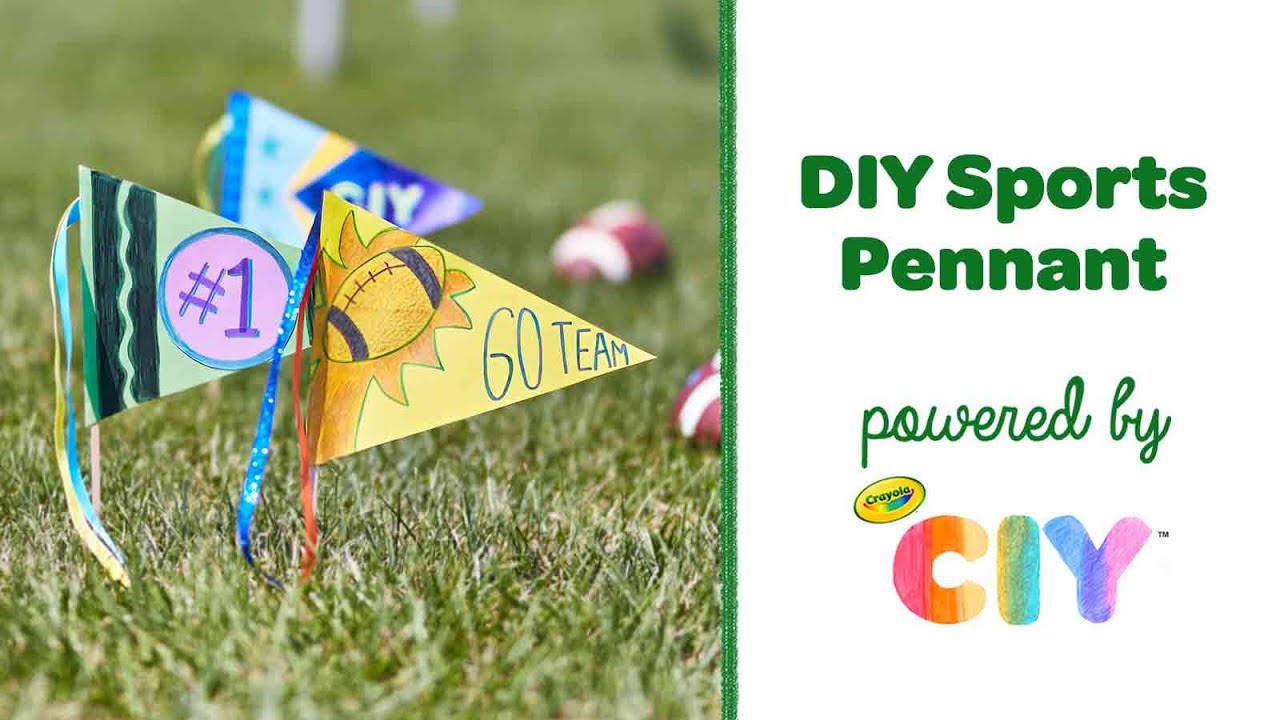The advertisement for a Crayola-powered DIY sports pennant project features a split-view image. On the right side, a white bar prominently displays the text "DIY Sports Pennant," followed by "powered by Crayola," both in dark green letters. The Crayola logo, set against a yellow backdrop, accompanies the multicolored, rainbow-like "C-I-Y" letters, indicative of the "Crayola It Yourself" concept.

On the left side, set against a vivid grassy background bathed in sunlight, three triangular paper pennants are clearly visible. The front pennant, bright yellow, reads "Go Team" in blue marker, adorned with an orange football and a dynamic swoosh. The middle pennant is green, featuring a purple circle with the text "Number 1." It has a darker green stripe on the left side. The third pennant in the background, primarily blue with a yellow and lighter blue swoosh, is marked with "C-I-Y" and includes a small, darker blue diamond. Also scattered on the grass are two footballs, one fully visible and the other partially cut off at the edge of the photo.